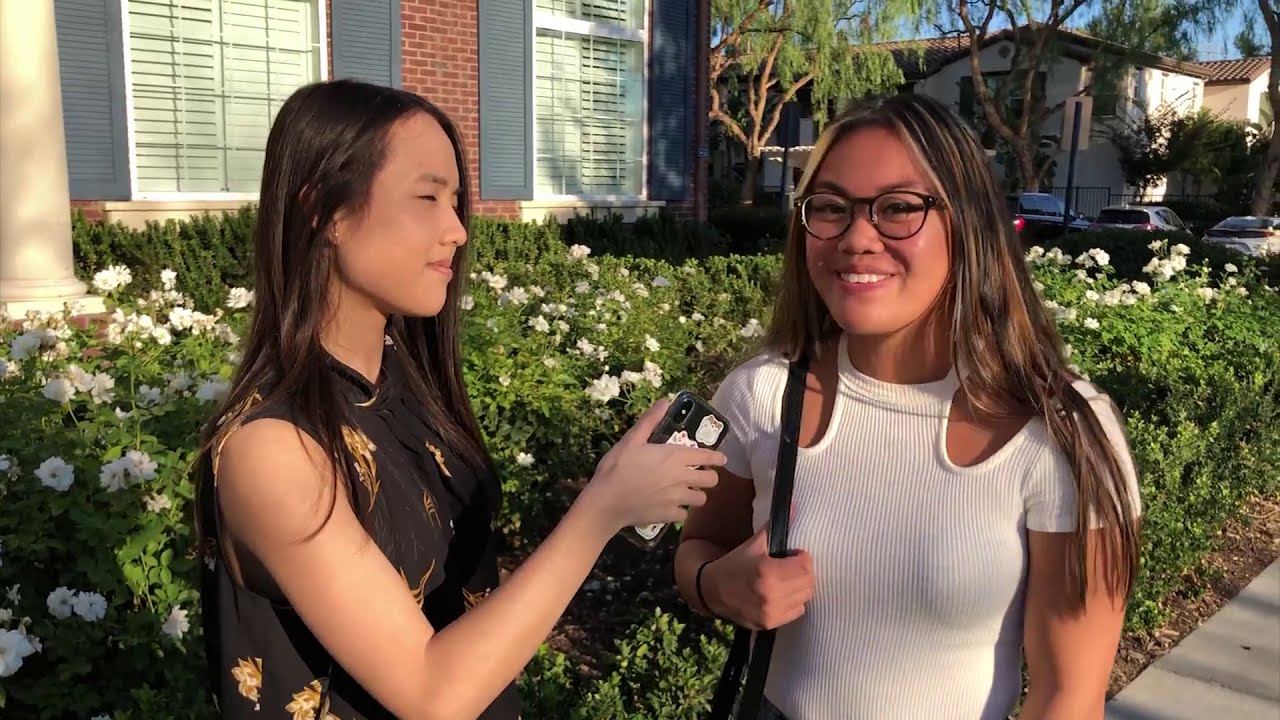A sunny outdoor scene captures two college-age women engaged in what appears to be an interview. Centered in the photo, the woman on the left has long black hair and wears a sleeveless black top adorned with gold floral designs. She is holding a phone up like a microphone with her right elbow bent, directing it towards the other woman. This second woman, who is facing forward and smiling as though speaking, has long brown hair streaked with blonde highlights. She wears circular black glasses and a white, short-sleeved shirt with cutouts around the shoulders. A purse hangs over her right shoulder. They stand on a sidewalk in front of a hedge with small white flowers, with a parking lot and several buildings, including a brick house with blue shutters, visible in the background. The bright sunlight makes the scene gleam, with both women squinting slightly due to the brightness.